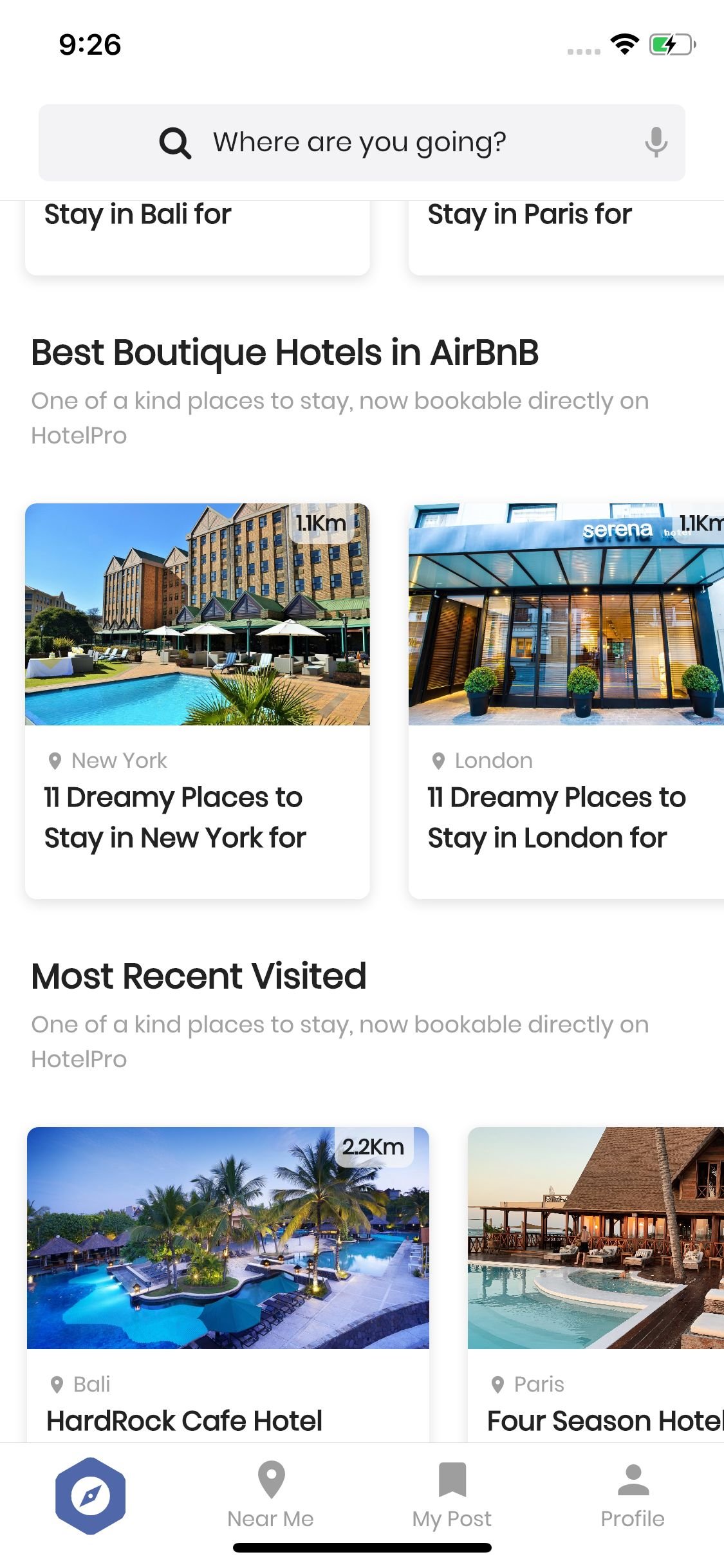This is a detailed screenshot of an Airbnb app interface. At the top of the screen is a white search bar with the placeholder text, "Where are you going?" To the left of the text is a magnifying glass icon, and to the right, a grayed-out microphone icon.

Below the search bar, there are two suggestion tags: "Stay in Bali" and "Stay in Paris." Further down, the display name on the page reads "Best Boutique Hotels in Airbnb," which introduces two featured articles. The first article, titled "11 Dreamy Places to Stay in New York," is highlighted on the left. To its right, another article titled "11 Dreamy Places to Stay in London" is featured.

The next section, labeled "Most Recently Visited," showcases two image bubbles. The first image bubble is a picture of the Hard Rock Cafe Hotel in Bali. The second image bubble features the Four Seasons Hotel in Paris.

The app's background color is predominantly white, including the header and footer sections. The footer contains four icons: on the far left is a hexagon icon shaded in periwinkle with a compass inside it, indicating the 'Explore' section. Next is the 'Near Me' icon, followed by the 'My Post' icon, and on the far right, the 'Profile' icon.